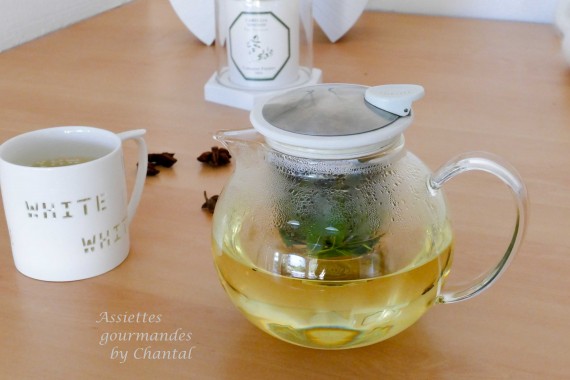This horizontal rectangular image captures a kitchen or countertop setting with a clear glass teapot and a white mug prominently displayed. The countertop is a light brown, possibly beige, and in the background, a white wall can be faintly seen where it intersects with the table. 

In the center of the image, the clear teapot contains a light amber-colored liquid, likely green tea. The teapot features a white top with a silver accent and a clear glass handle. To the left of the teapot is a white mug with the word "white" printed twice in gray letters. 

Behind these items, a partly visible white object with a dark gray hexagram design can be seen. Spread around the top of the countertop are some indeterminate black objects. In the bottom left corner of the image, white text reads "Asiats Gourmandis by Chantal."